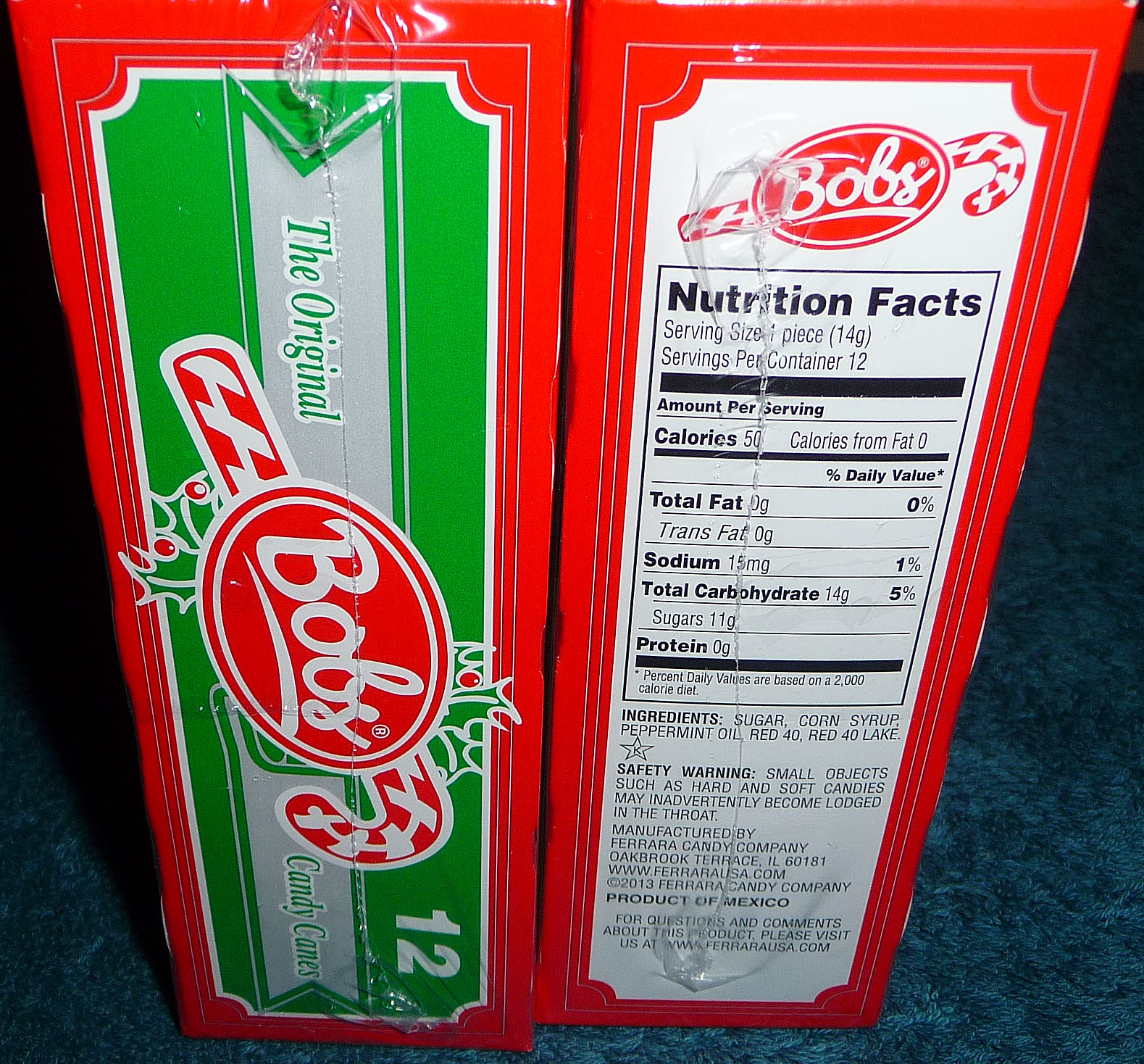The image features two vertically rectangular boxes of Bob's Candy Canes, displayed side-by-side on a dark blue background that appears to be some sort of fabric. The left box is primarily red with a large green rectangle in the center, overlaid by a gray vertical stripe, bearing the words "The Original Candy Canes" in green. A red and white candy cane, accented with green holly and red berries, is placed diagonally across this stripe, along with a red oval containing the word "BOB'S" in white. The number 12 appears in white at the bottom of the green rectangle, indicating the quantity of candy canes.

The right box shares the same red border but has a large white section in the center. This side also features the red and white candy cane with the "BOB'S" logo, oriented horizontally this time. Below this, in black and white, is the nutrition facts panel detailing calories, total fat, sodium, carbohydrates, protein, and includes ingredients and safety warnings. Both boxes are sealed in plastic wrap. The image is taken from a slightly downward angle, providing a clear view of the product's packaging and branding from different perspectives.